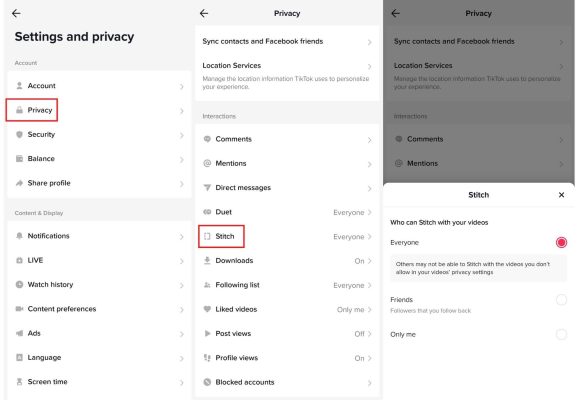The image displays three different screenshots representing various sections of the settings and privacy options. Each section is navigated by a back arrow at the top, indicating they may be separate screenshots. 

In the first section titled "Settings and Privacy," the "Privacy" option is prominently highlighted with a red box. This section lists various options including Account, Privacy, Security, Balance, and Share Profile.

The second section dives deeper into privacy settings and contains a variety of options such as Sync Contacts, Facebook Friends, Location Services, Comments, Mentions, Direct Messages, Duet, Downloads, and Following List. Here, the "Stitch" option is notably highlighted in red. 

The third section focuses specifically on the "Stitch" setting. On the right-hand side of the screen, about halfway down, it shows that the "Who can stitch with your videos" setting is toggled on "Everyone". Above this segment, the top of the page is shaded gray, indicating the heading "Sync Contacts" from an earlier screen.